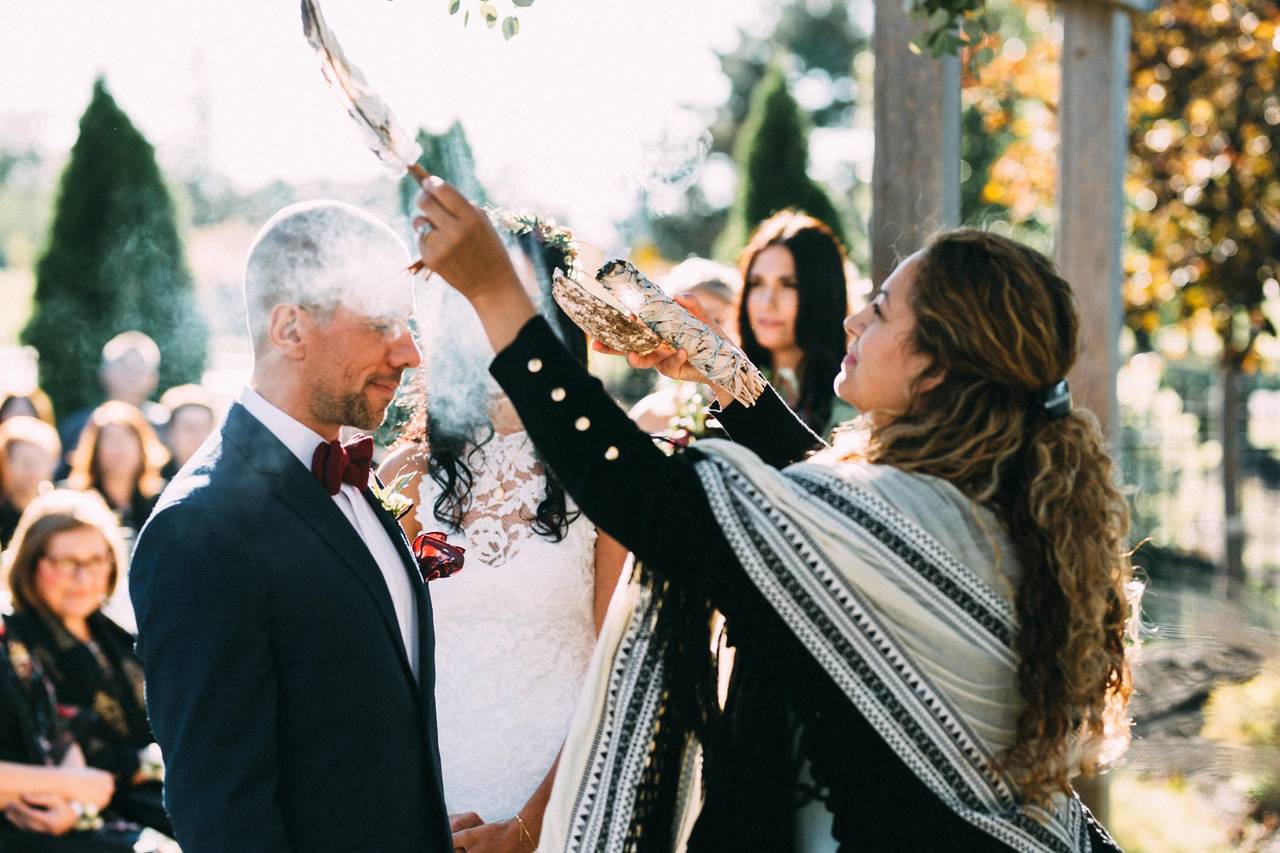In this evocative image of a smudging ceremony at an outdoor wedding, attendees can be seen seated in the background amidst a setting adorned with lush trees, bushes, and elegant columns, highlighting the natural beauty of the environment. The focal point is a woman, likely in her 30s or 40s, with long, thick, wavy hair that is predominantly a dark shade of brown, accentuated with blonde highlights. She is draped in a striking, long cloak that features a white and gray palette with intricate patterns of triangles, dots, and lines, paired with a black long-sleeved top underneath. In a moment of spiritual cleansing, she holds an eagle feather in her left hand and sage in her right, as she gently smudges the groom—a young white man in his 20s—who is dressed impeccably in a black tuxedo and red bow tie, his short hair neatly groomed, and his beard and mustache well-trimmed. The bride, with flowing dark brown or black hair that extends past her shoulders, stands beside him in a beautiful white bridal gown. Although her face is not visible, the serene and sacred atmosphere of the smudging ceremony, set against the backdrop of an outdoor wedding, is palpable.